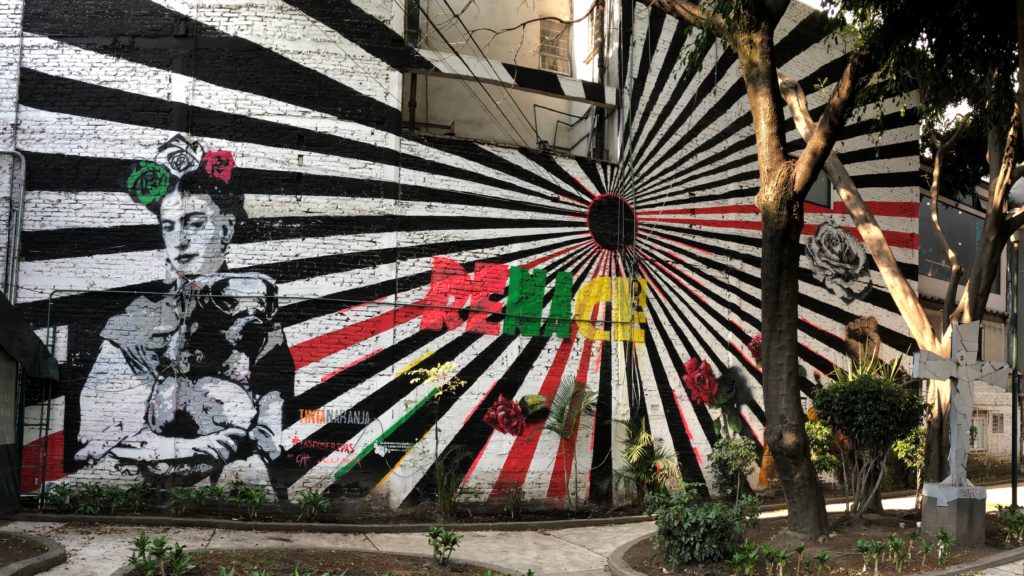This photograph captures a vivid mural painted on the side of an old, whitewashed brick building during the daytime, possibly at sunset during the golden hour. The mural's central feature is a black sun resembling the imperial flag of Japan, with most of its radiating beams in black and five beams distinctly in red. In the center of this rising black sun is the word "RENACE," with "R-E" in red, "M-A" in green, and "C-E" in yellow.

To the right of this striking pattern is a detailed black and white drawing of a blooming rose, below which is a powerful raised fist symbolizing resistance or solidarity. On the left side of the mural is a black and white portrayal of Frida Kahlo. She stands solemnly with three flowers in her hair—one red, one white, and one green—representing the colors of the Mexican flag. In her arms, she cradles a dog that appears to be the famed earthquake rescue dog, distinguishable with its goggles.

Below the mural, the sidewalk leads past some bushes and a tree situated in a small planting area, along with a prominent stone cross suggesting a possible religious or memorial significance. The artist's signature is visible in orange and gray letters, though it is not entirely legible. This mural combines vibrant colors, historical reference, and poignant imagery to create a compelling outdoor artwork.